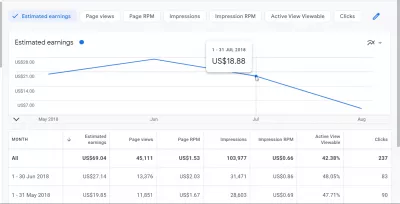Screenshot of a webpage featuring analytics with a chart and a table:

At the top-left corner, there's a section labeled "Estimated Earnings" accompanied by a blue checkmark and blue text. To the right of this label, there are six white buttons: "Page Views," "Page RPM," "Impressions," "Impressions RPM," "Active View Viewable," and "Clicks." Adjacent to these buttons is a blue pencil icon.

Beneath this section is a chart also titled "Estimated Earnings." At the center of the chart, there is a pop-up window displaying the earnings amount, which is USD $18.88. 

Below the chart, there’s a detailed table with eight columns, presumably listing metrics related to the chart data.